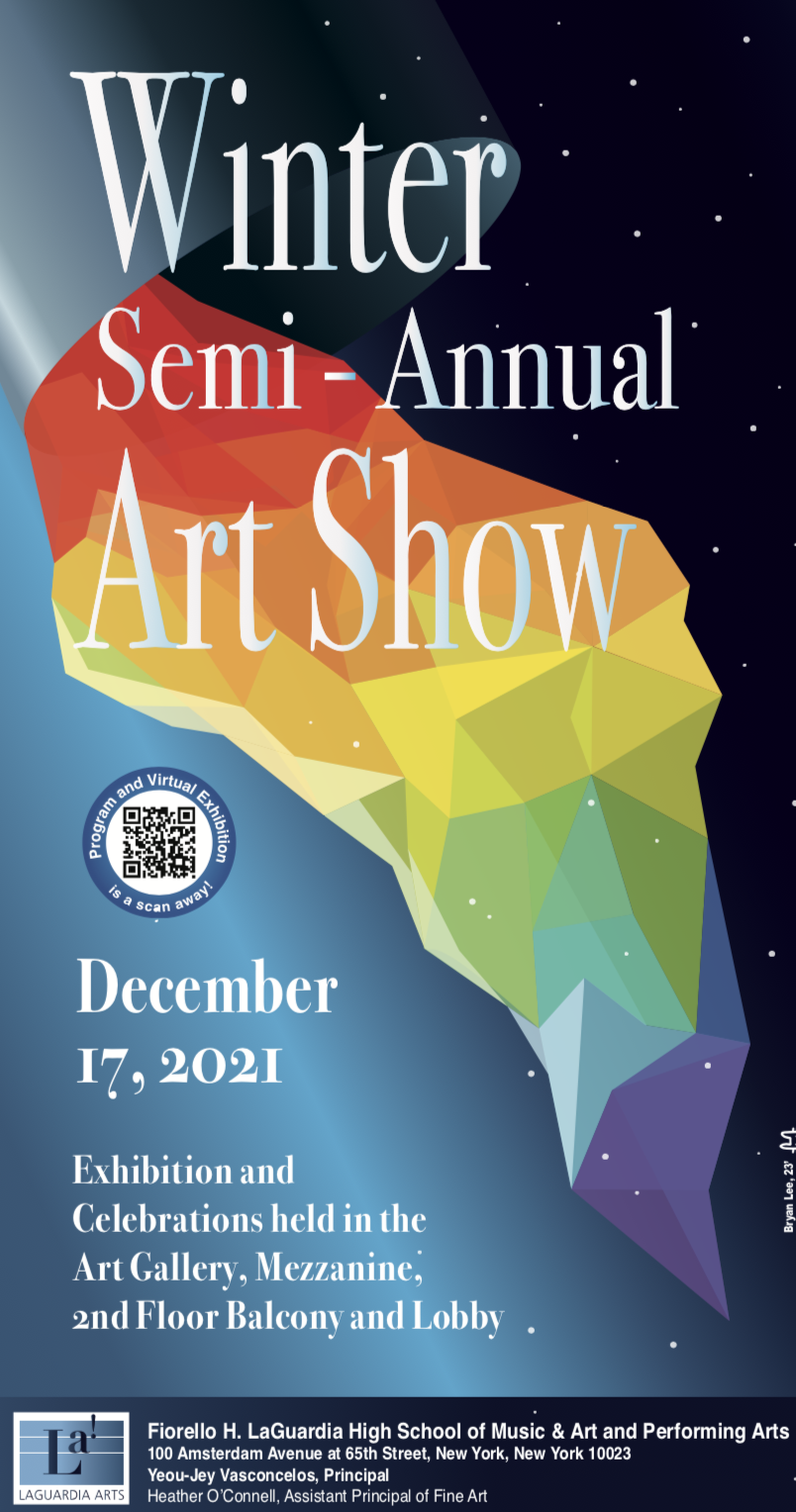The poster advertises the "Winter Semiannual Art Show" scheduled for December 17, 2021. The event will feature exhibitions and celebrations held in the art gallery, mezzanine, second floor balcony, and lobby. The poster's background merges a night sky with twinkling stars on the top left into a silverish-blue nebula-like design. A striking multicolored crystal sits in the center, displaying hues of red, orange, yellow, light blue, dark blue, and purple. A QR code in the middle of the poster likely directs viewers to more information or ticket options. Additional details, including the event's specific location and address, are provided at the bottom. The overall design is vibrant and illustrated in a cartoon-style manner with a vertical split in color themes—blue on the left and starry black on the right.